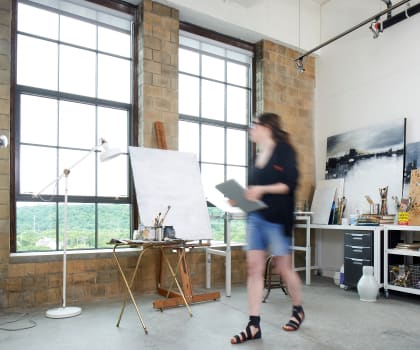In the photograph, a spacious, light-filled artist studio is captured with meticulous detail. To the left, a light brown brick wall supports nearly floor-to-ceiling windows adorned with a checkered grid, allowing ample natural light to flood the room. The windows extend almost to the ground, creating an open and airy atmosphere. The studio's cement floor adds to the industrial feel, while the large white wall in the background contrasts with the brick.

In the center of the room, a woman is captured mid-motion, resulting in a slightly blurry image that partially obscures her identity. She has brown hair and wears a black top and jacket, blue cut-off jeans, and black gladiator sandals. Clasped in her hands appears to be a music book or an art folder, adding to the creative ambiance. She glances over her shoulder as if in thought, immersed in her environment.

Surrounding her, the studio is brimming with artistic essentials. A large brown easel stands prominently with a hefty white notepad attached, ready for the next masterpiece. Various painting canvases are scattered around, and a desk cluttered with art supplies hints at the ongoing creation process. In the background, a completed white and gray painting of a serene lake scene hangs, adding a finished touch to the workspace. The overall atmosphere suggests a dynamic and inspiring setting where art and creativity flourish.